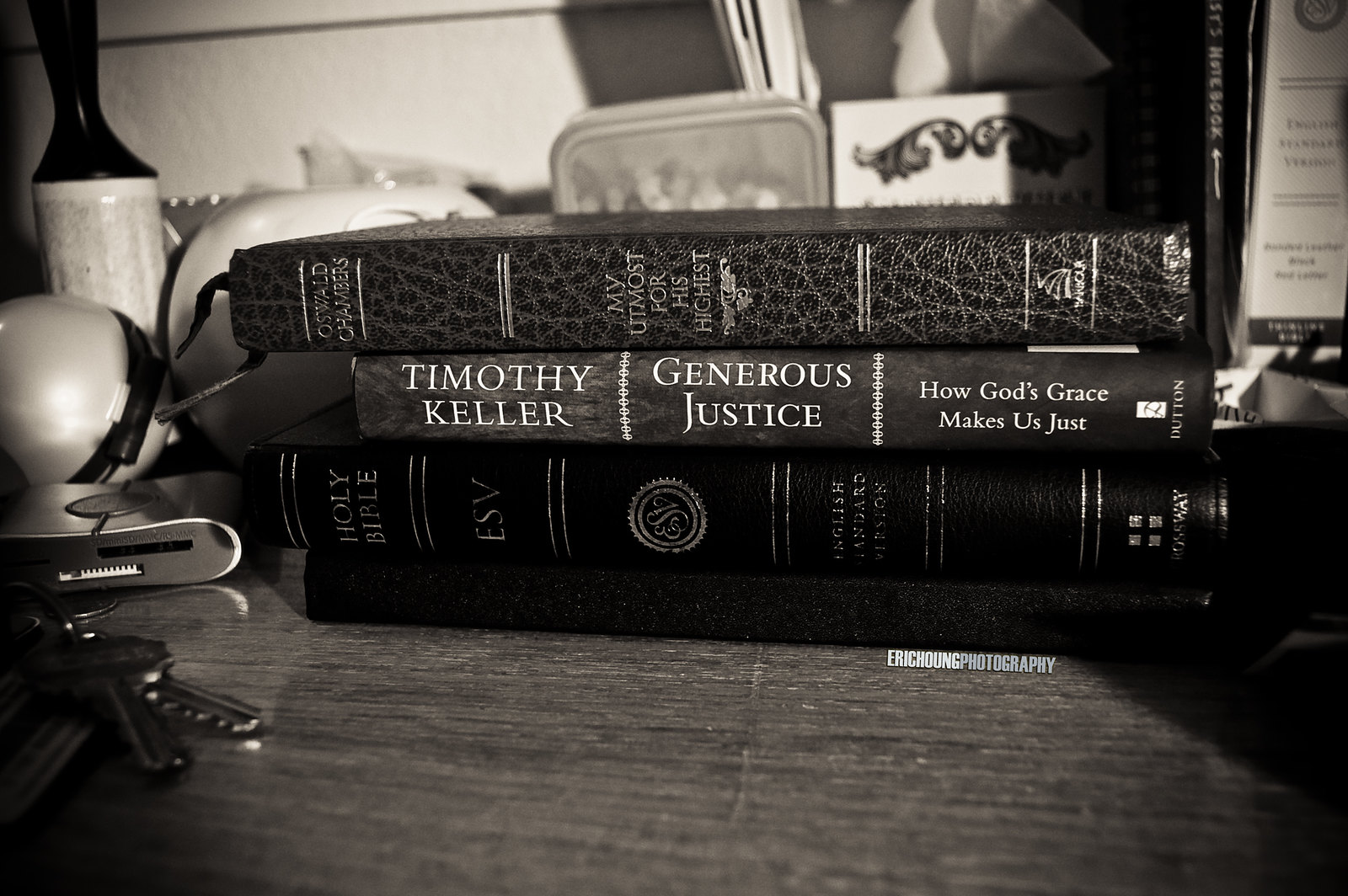The monochromatic photograph captures a close-up view of a wooden table laden with various items. Central to the scene is a neatly stacked arrangement of four books, their spines facing the camera. Dominating the pile is "My Utmost for His Highest" by Oswald Chambers, with its elegant binding featuring some delicate decorative elements. Below it sits "Generous Justice: How God's Grace Makes Us Just" by Timothy Keller, clearly identified with its neatly embossed title and author's name in capital letters. Nestled second from the bottom is "The Holy Bible," distinguished by its classic typographic design and decorative lines. The final book at the base remains nameless, with minimalistic writing barely visible on its lower right corner.

Beyond the books, the table hosts an assortment of everyday items, including a set of keys, what appears to be a lint roller, a cell phone, and other miscellaneous objects like tissues and cards. The background hints at additional framed items or decorative pieces against the white wall. Together, the objects weave a narrative centered on Christianity, suggesting the personal nature of the collection captured in this timeless black-and-white moment.